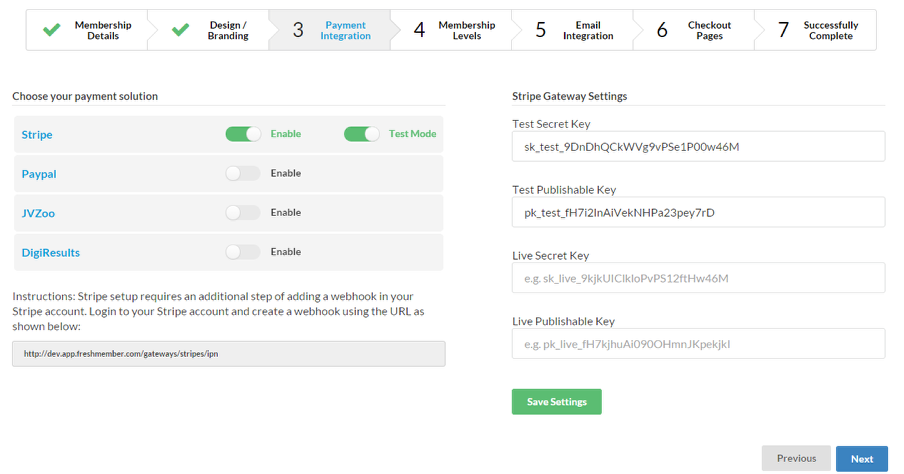This screenshot captures a detailed view of a web page, showcasing a comprehensive interface for managing membership and payment integrations. 

**Header Navigation:**
At the top of the page, a horizontal menu bar includes several options: 
- Membership Details
- Design Branding
- Payment Integration
- Membership Levels
- Email Integration
- Checkout Pages
- Successfully Complete

**Left Pane: Payment Solutions:**
On the left side, there is a section where the user can select from different payment solutions. Each option features a toggle switch to enable or disable the service. The available payment solutions are:
- Stripe (currently enabled in test mode)
- PayPal
- JV Zoo
- DigiResults

**Right Pane: Stripe Configuration:**
On the right side of the page, there are four text entry fields for configuring the Stripe payment gateway. These fields are labeled as:
- Test Secret Key
- Test Publishable Key
- Live Secret Key
- Live Publishable Key

Each field is ready to accept the respective API keys necessary for integrating and testing the Stripe payment provider in both test and live environments.

This screenshot likely serves as an administrative interface for managing payment settings and account configurations seamlessly.